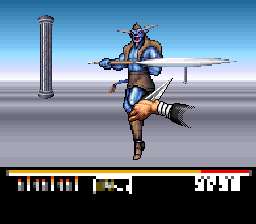This image appears to be a screenshot from a vintage turn-based role-playing video game, reminiscent of classics like Final Fantasy. The central figure is a blue-skinned, horned creature, possibly an alien or robot enemy, facing slightly to its right. The character, who has a tail, wears a brown cap and has brown fur or clothing draped over its shoulders, with a matching loincloth or skirt and brown boots. The creature is depicted in a dynamic stance, balancing on one leg while holding a sword horizontally. One hand grips the hilt, while the other hand is bent upwards, holding the blade. The background features a gray floor with a distinct pillar nearby and another further back, all under a blue sky. Additionally, there's a disembodied hand, possibly the player's character, holding a knife at the bottom of the image. There is a colorful interface at the bottom, consisting of a yellow and white bar merged with red and white, flanked by gray ends, and various dash-like symbols in gray, red, white, and olive green.